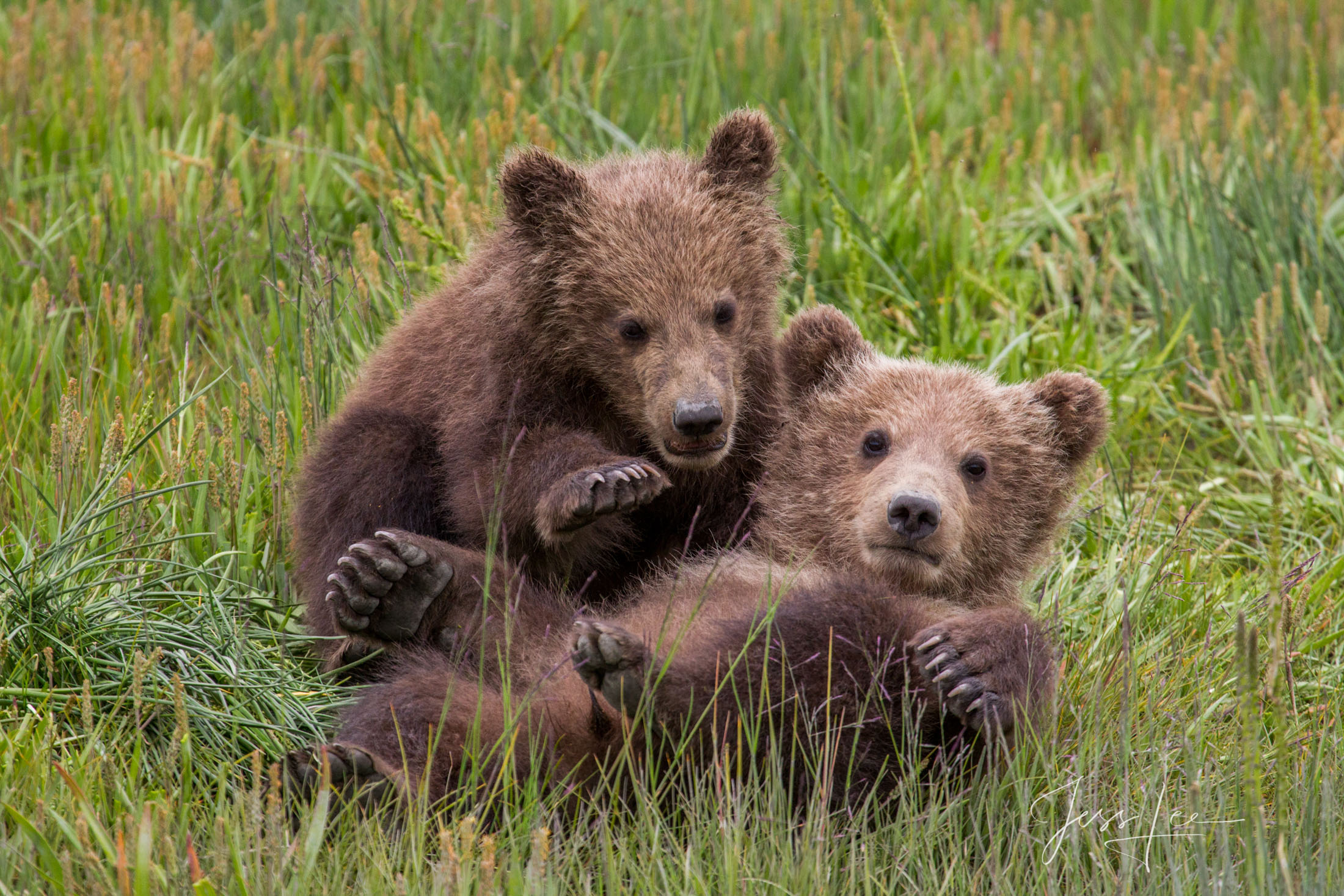This is an incredibly detailed, crisp photograph showcasing two adorable baby brown bears playing in a field of tall green and brown grasses. The bear on the left is in a crouched position, lightly hovering over its sibling who is lying on its back, legs in the air, almost as if being embraced. They both have light brown, bristly fur and sharp claws, with one bear’s paw raised and the pads of a foot clearly visible. Their expressive faces are captured perfectly as they seem to be looking directly into the camera, drawing the viewer in with their cuteness and curiosity. This image, possibly a highly realistic digital creation or an expertly timed photograph, features the artist's signature, "Jess Lee," in delicate white cursive in the corner.